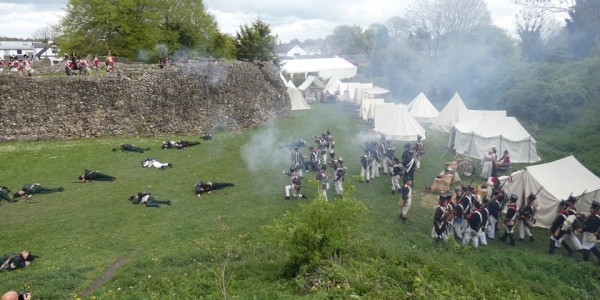This detailed color photograph captures a vivid Revolutionary War reenactment scene set in a lush, green landscape surrounded by trees and sporadic shrubs. The focal point is a sprawling grassy field, where both American and British reenactors are engaged in an intense mock battle. On the left, a stone wall that resembles a fortification extends upward, with spectators and a few drummers positioned atop it. In the field below, some soldiers lie motionless, simulating casualties of a recent skirmish.

The American soldiers, positioned predominately in the lower right of the image, are dressed in historically accurate uniforms consisting of white pants, dark blue overcoats, and black boots. Opposing them, in the upper left section of the image, are the British soldiers, distinguishable by their iconic red coats. Both sides wield long muskets, with visible plumes of smoke billowing from the barrels, indicating recent discharges of gunfire.

The encampment is filled with numerous white canvas tents scattered across the grass, creating a vibrant backdrop of 18th-century military life. Among the encampment, women in long dresses add to the period atmosphere, though they appear distant and somewhat detached from the immediate drama of the battlefield below. The overall scene is bustling with reenactors and spectators alike, vividly recreating a historical clash amid the verdant, lively landscape.